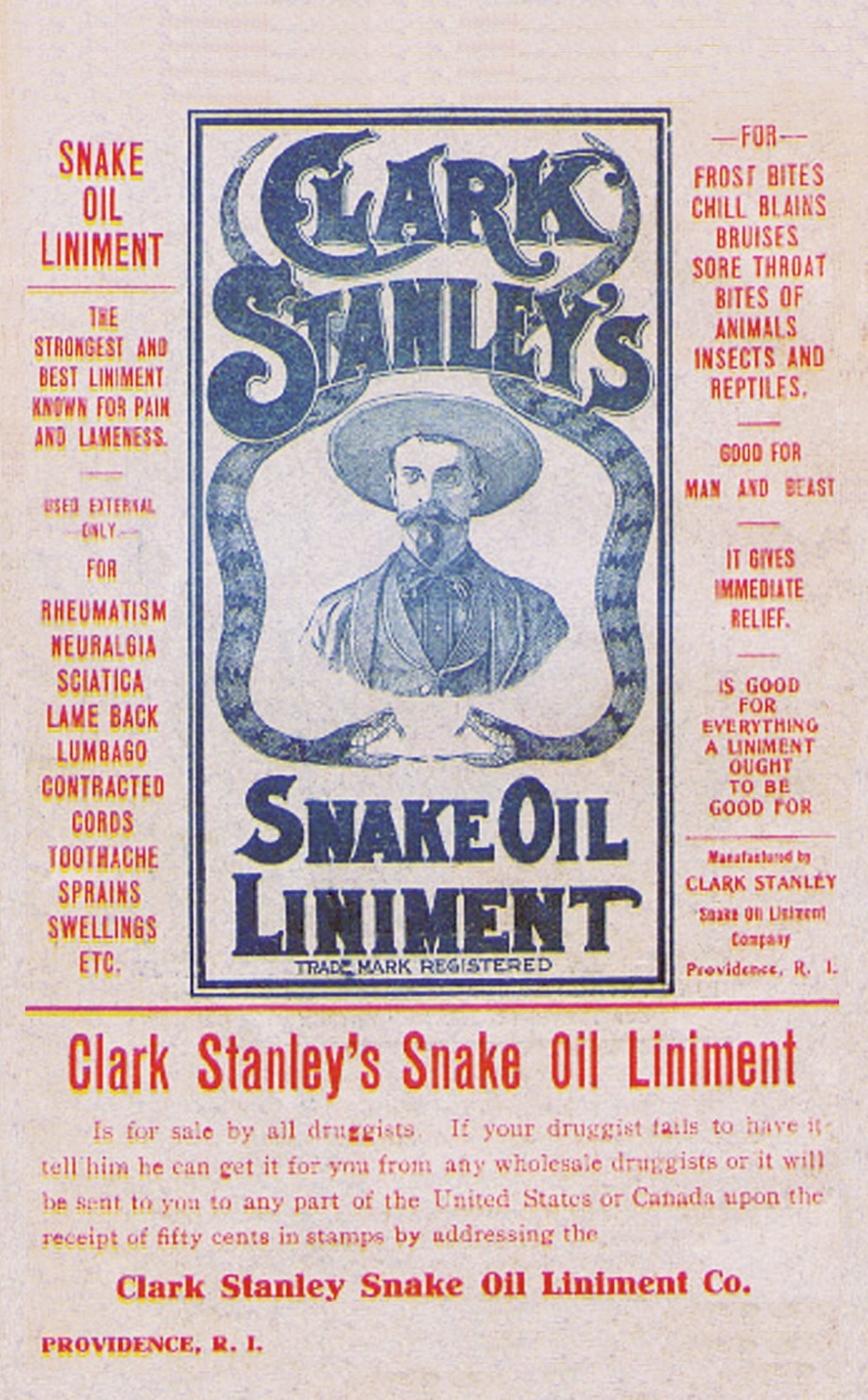This color photograph captures a detailed and well-preserved advertisement for Clark Stanley's Snake Oil Liniment, styled to resemble a 19th-century promotional piece. The background is a pale beige, potentially indicating a modern reproduction of the old-fashioned ad. Central to the image is a rectangular box featuring a striking illustration of Clark Stanley dressed in a cowboy hat, goatee-type beard, mustache, coat, and vest. Flanking Stanley are two ominous-looking snakes with their fangs bared, positioned as if facing each other, possibly with venom or snake oil depicted as dripping from their mouths.

Prominent blue text in the middle announces "Clark Stanley's Snake Oil Liniment," while surrounding red text provides various claims about the product's effectiveness. This liniment is touted as the strongest and best known for alleviating pain and lameness. It claims to treat a myriad of conditions including rheumatism, neuralgia, sciatica, lumbago, lame back, toothaches, sprains, swellings, frostbites, chillblains, bruises, sore throats, and bites from animals, insects, and reptiles. Additional bold claims state that it is beneficial for both man and beast, offering immediate relief for everything a liniment ought to address.

At the bottom of the advertisement, more information includes pricing and availability: "Manufactured by Clark Stanley's Snake Oil Company, Providence, Rhode Island." It specifies that the product is available at all druggists and can be directly ordered from any part of the United States or Canada for 50 cents in stamps. This richly detailed advertisement provides a glimpse into the historic marketing of patent medicines, complete with grandiose claims and vivid illustrations.